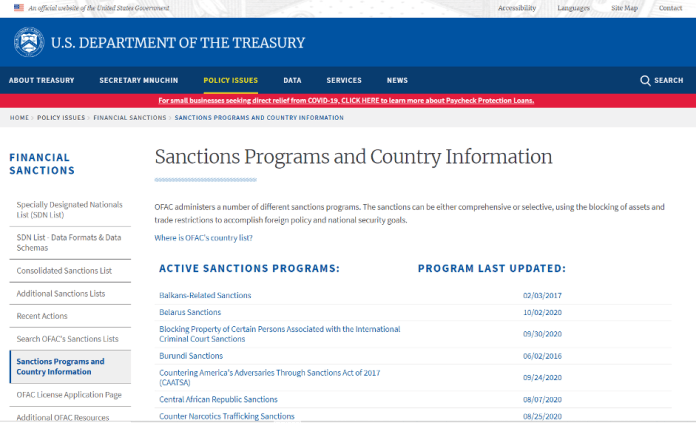This image is a detailed screenshot set against a white background. In the upper-left corner, there is a small icon of the American flag, symbolizing the national identity of the organization. The upper-right corner features navigation tabs labeled "Accessibility," "Languages," "Sitemap," and "Contact," providing users with essential website functions. 

A prominent blue banner beneath these options displays the title "U.S. Department of the Treasury," indicating the official nature of the site. Directly below, a darker blue banner with white text includes various navigation options: "About Treasury," "Secretary Newton," "Policy Issues," "Data," "Services," and "News," allowing users to explore different segments of the department's offerings.

A narrow red banner follows, aiming to assist small businesses impacted by COVID-19. It reads, "For small businesses seeking direct relief from COVID-19, click here to learn more about Paycheck Protection Loans," offering a direct link to resources and support.

Below the red banner, against the same white background, there is a section titled "Sanctions Programs and Country Information." It explains that the Office of Foreign Assets Control (OFAC) administers various sanction programs. These sanctions can be either comprehensive or selective, utilizing asset blockages and trade restrictions to fulfill U.S. foreign policy and national security objectives.